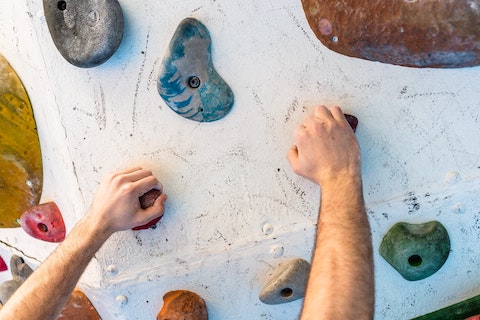A climber's forearms stretch out, fingers clutching onto the vibrant synthetic rock holds strategically positioned on the climbing wall. The wall's surface is a canvas of mars, scrapes, and scuffs, evidence of previous climbers’ grit and determination. The holds, kidney-shaped and adorned in a spectrum of colors, provide essential grips with their tiny indentations. Against a stark white background, these holds, each bolted securely into place, form a challenging path. In the upper right corner, a larger hold contrasts the smaller, scattered handholds below. The scene captures the raw intensity of the climb, with each mark on the wall narrating a story of past ventures.